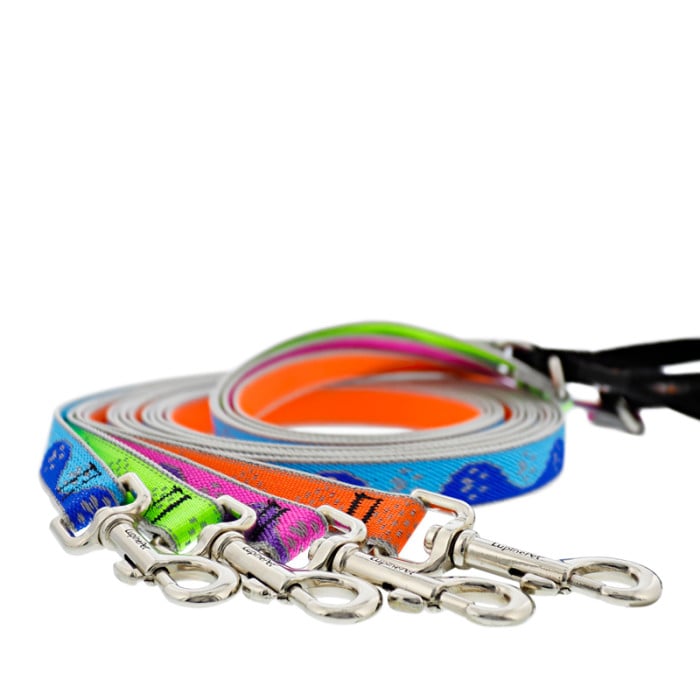This color photograph features a tightly coiled grouping of four dog leashes, each with a silver metal clip at the end. The leashes are wrapped together in a circular fashion, with the clips prominently displayed in the foreground. The vibrant leashes include a blue one with an interlocking wave pattern of royal and light blue with gray speckles, a lime green one, a fuchsia pink one with purple accents, and an orange one. Each leash, predominantly the neon color corresponding to its primary hue, forms a concentric circle with gray edges visible at the top of the loop. The coiled leashes appear to be connected to black straps or an object at one end. The background of the image is plain white, emphasizing the colorful arrangement and clean appearance of the neatly organized leashes.